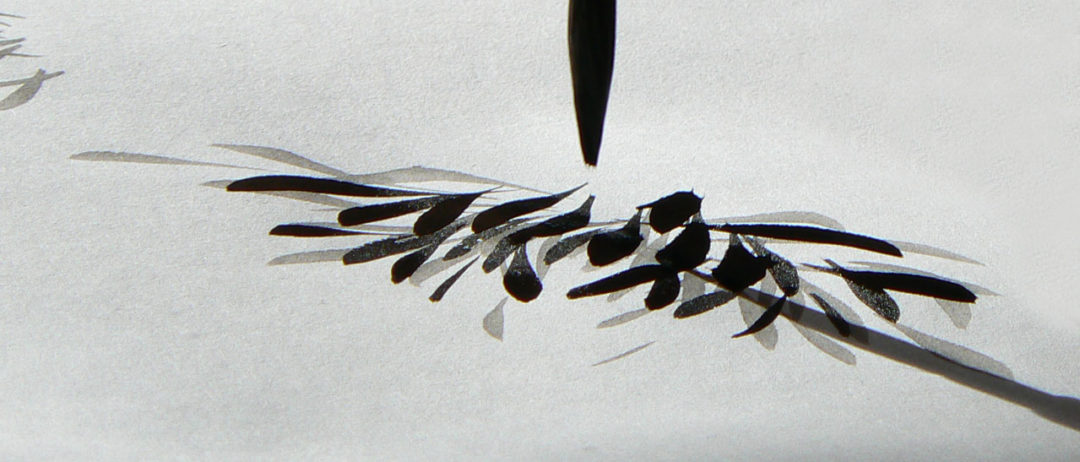This black-and-white abstract image, resembling a blend of Chinese watercolor painting, ink drawing, and representationalism, depicts a striking floral theme. At the center, abstract leaf-like structures dominate, primarily in dark black hues with gray shadows beneath them. A solid black brush tapers from the top center to the middle, resembling an ink pen or paintbrush, suggesting artistic creation in progress. The composition is concentrated mainly toward the right side and center, with some sparsely placed gray leaf-like forms on the left. A branch originates from the right, curving inward. The background, a dull light gray, enhances the stark contrast of the black and gray markings, giving the image a cold and stiff appearance. The entire piece, devoid of geometric forms and text, evokes a somber yet intricate floral narrative.